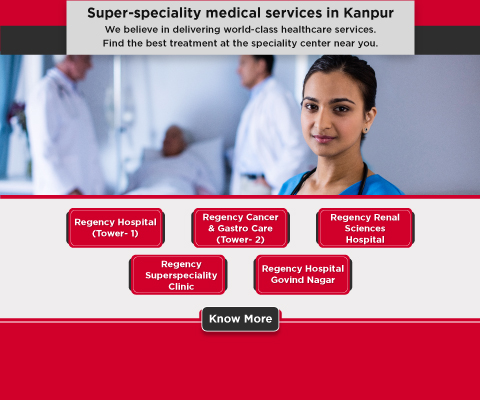The image features an advertisement for medical services in Kanpur. At the top, a white dropdown box with black font reads, "Super Speciality Medical Services in Kanpur. We believe in delivering world-class health care services. Find the best treatment at the specialty center near you." Flanking the dropdown box are red and black stripes on either side. Below this, a professional photograph depicts an Indian woman dressed in blue scrubs with a stethoscope draped around her neck, identifying her as a nurse. She is looking directly at the camera and wearing earrings. In the background, a patient lies in a hospital bed, attended by two doctors in white lab coats.

Beneath the image, there is a white box containing a list of facilities represented by red-highlighted labels: Regency Hospital (Tower 1), Regency Center and GastroCare (Tower 2), Regency Renal Sciences Hospital, Regency Super Speciality Clinic, and Regency Hospital, Govind Nagar. At the bottom of the advertisement, a black button with white text reads "No More," and this is set against a solid red box. The entire advertisement is set on a white backdrop, reinforcing its professional and clean design.